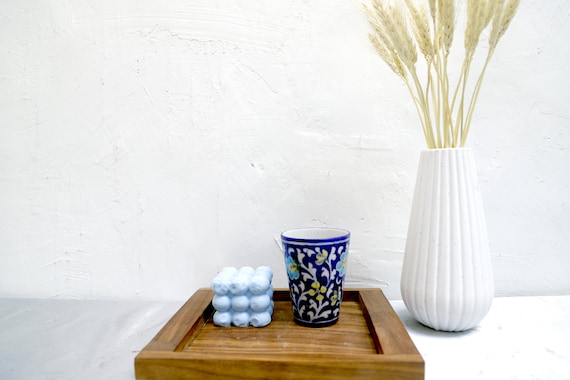The photograph displays a square wooden serving tray positioned on a white to grayish granite-finished countertop, likely in someone's kitchen or home. The tray, crafted from a warm brown wood, features a blue and white ceramic cup adorned with intricate hand-painted floral patterns. Adjacent to this cup, on the left side of the tray, is a small stack of what appears to be ice cubes in a clear glass or a decorative cube made of little blue balls. To the right of the serving tray stands a six-inch tall, round white vase, which tapers upwards and contains several stalks of tall brown wheat with grain tops. The entire setup is set against a pristine white wall, creating a clean and elegant backdrop for the decorative arrangement.